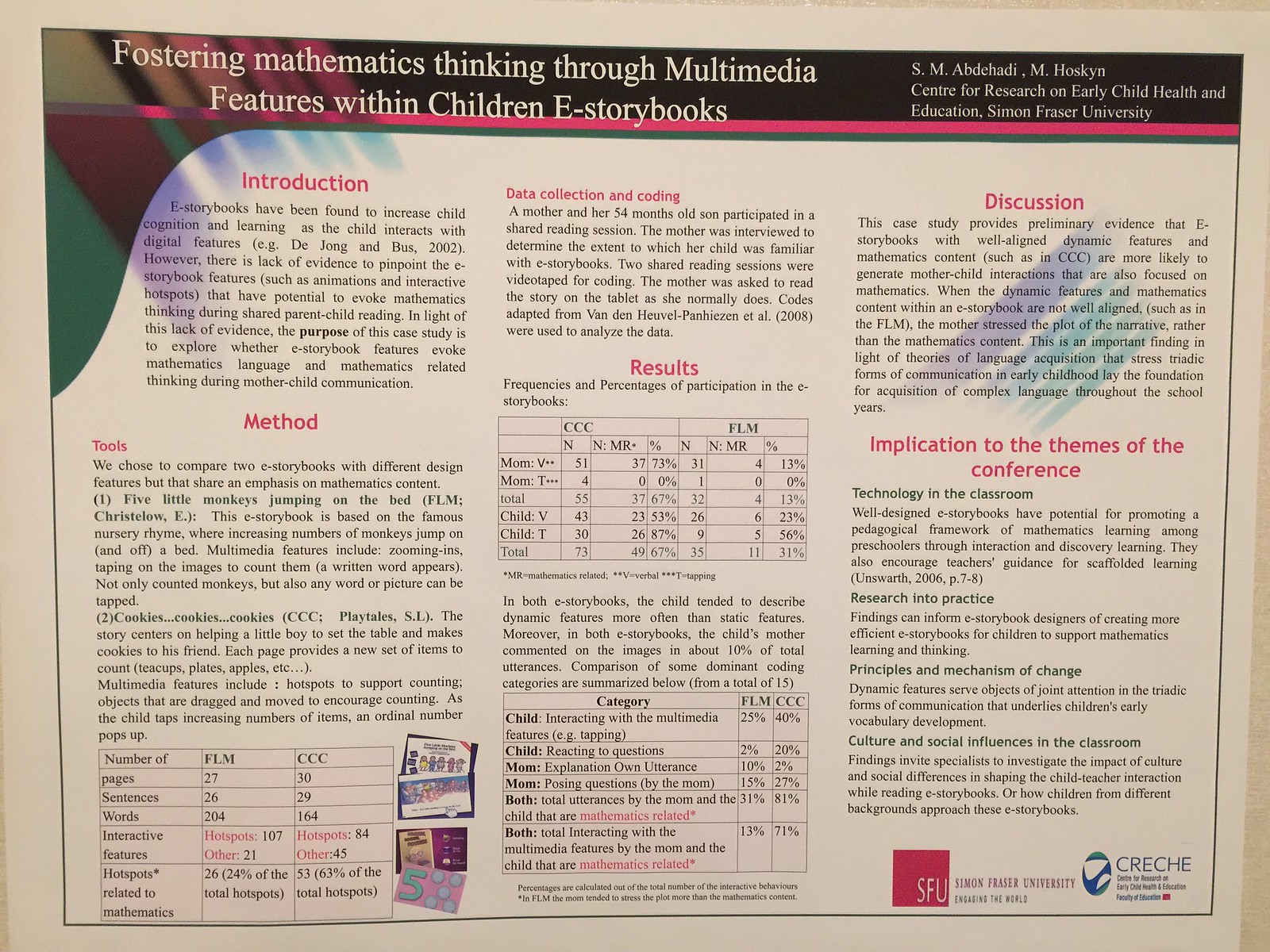The image displays a densely information-packed poster board, likely from an academic or classroom setting. Centrally positioned within the image, this sheet prominently features a colorful banner at the top, adorned with shades of light violet, light blue-green, red, dark green, burgundy, pink, and hot pink. The banner bears the title "Fostering Mathematics Thinking Through Multimedia Features Within Children eStorybooks" and includes the credentials "S.M. Abduhadi and M. Hoskin, Center for Research on Early Child Health and Education, Simon Fraser University" on the right.

The main body of the poster is divided into three columns of information. Starting from the top left, the sections are detailed as follows: "Introduction," followed by "Method." The middle column headings in red include "Data Collection and Coding" and "Results," which also presents various data tables. The right column features the sections "Discussion" and "Implication to the Themes of the Conference." The colors black and white provide a clear contrast for the text, making it distinct and organized. The overall setting of the poster suggests it is part of an educational display, potentially within a research-based context on early childhood mathematics and multimedia learning.